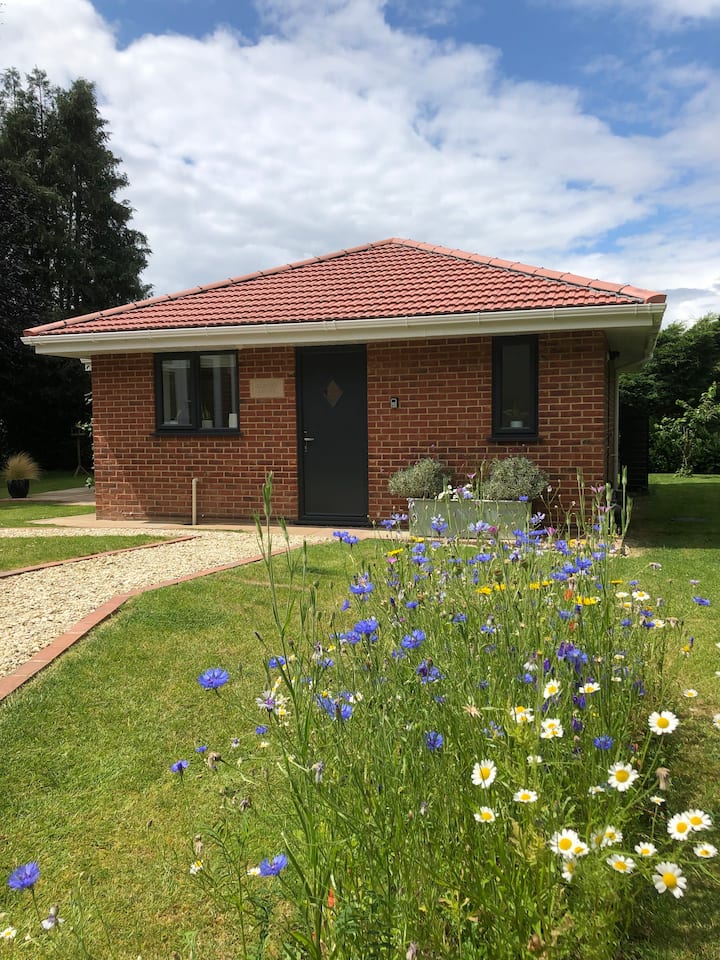This image showcases a small, traditional brick home with a distinctive Spanish tile roof characterized by its vibrant red hue. The house features a black metal door and three windows, two on the left side and one on the right, all adorned with black trim. The foreground highlights a meticulously mowed green lawn adorned with an array of plants and blooming flowers, including blue and white daisies with yellow centers. A gravel driveway slash walkway leads you to the door, flanked by a raised flower bed with bushes against the wall. Other green trees and plants in the background enhance the lush, verdant landscape surrounding the charming home.